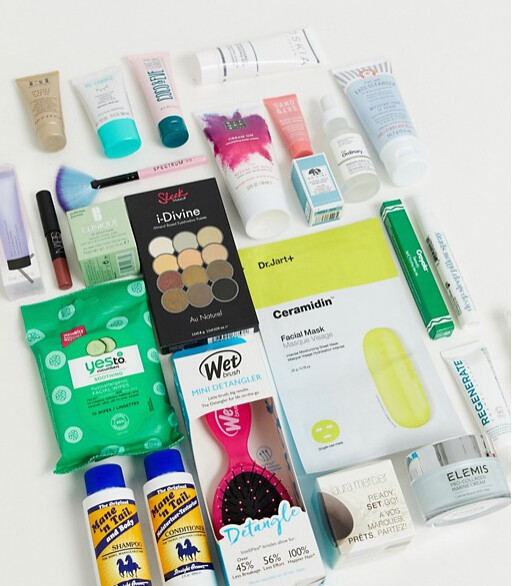A meticulously arranged composition of various skincare and beauty products against a pristine white background. The assortment includes a variety of packaging styles, from rectangular containers to cylindrical bottles. Prominently displayed in the center is a rectangular container of ceramide and facial mask, accompanied by a pink, wet-branded hairbrush. To the left of this are "Yes To" green face wipes, adding a touch of color to the left side of the image. Also in the center but slightly to the left is a sleek palette of eye shadow in a range of tan nudes to darker browns, labeled as "Divine Makeup." At the top right corner, one can spot ordinary dropper bottles, typically used for liquid skincare products. Other items include cylindrical bottles typical of face wash or beauty products, as well as a variety of rectangular packages and hairbrushes, ensuring a comprehensive showcase of skincare essentials.